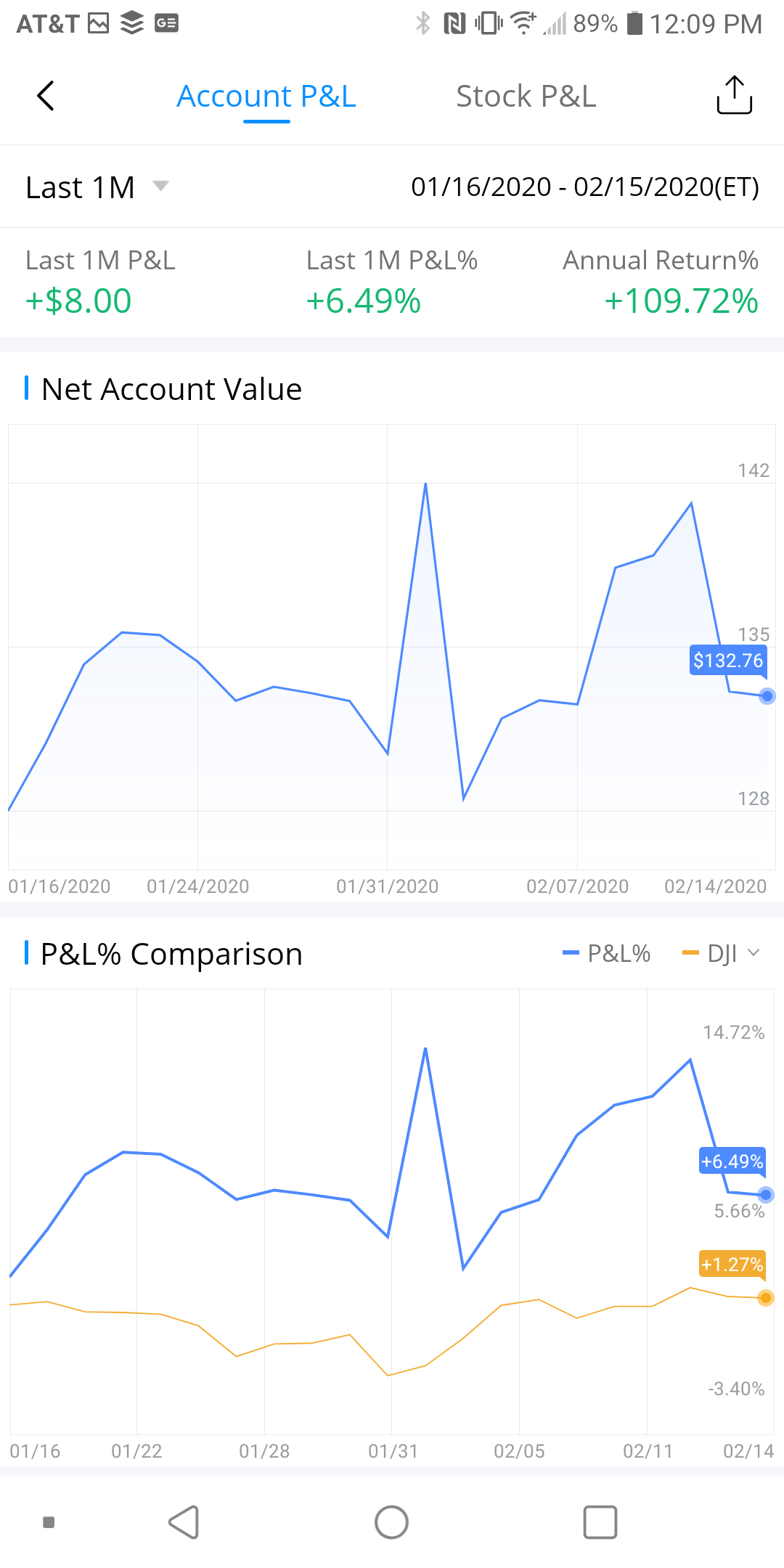Here is a cleaned-up and detailed caption based on the given information:

---

The screenshot captures the interface of a financial app, highlighting the “Account P&L” and “Stock P&L” tabs at the top center of the screen. The “Account P&L” tab is selected, indicated by a light blue color and a small blue line underneath it. Below these tabs, the main content area displays two centered line graphs. 

The top graph is titled "Net Account Value" and features a single blue line charting the value changes over time. The bottom graph, labeled "P&L Comparison," contains two lines: a blue line and an orange line running below it, comparing different P&L metrics.

Underneath the graphs, several performance metrics are displayed. The first metric, labeled "Last 1M P&L," shows a green figure of "+ $8." Next to it, another “Last 1M P&L” metric indicates a green percentage of "+ 6.49%.” The final metric on the right, titled "Annual Returns Percent," reports a green figure of "+ 109.72."

At the very bottom of the screen, the user's phone navigation icons are visible: a left-pointing arrow for back navigation, a circle for the home screen, and a square for recent apps.

---